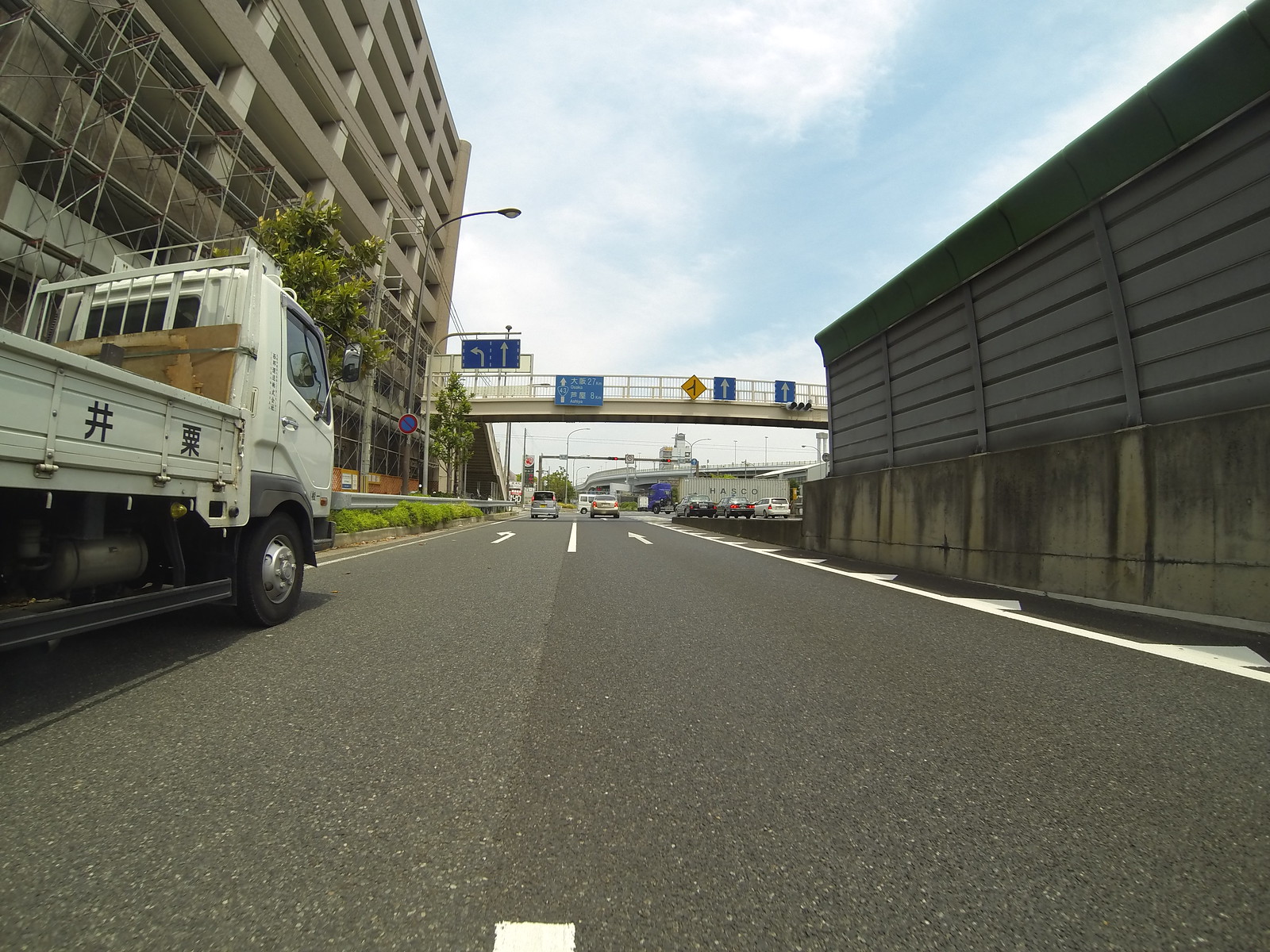This image, seemingly captured from the dash cam perspective of a car, showcases a detailed urban road scene. The road ahead is a dark grey with white lane markings, and a pedestrian bridge crosses overhead, featuring blue directional signs with arrows pointing left and straight ahead. The sky above is partly cloudy with a patch of blue visible to the right.

On the right-hand side of the road is a grey cement barrier with a darker grey metal fence atop it, potentially serving as a sound barrier. To the left, there is a white truck with potentially Japanese or Chinese characters and metal bars behind its cab. Further left, a tall building with scaffolding stands adjacent to a multi-level grey parking structure. 

Towards the front, traffic is visible in the distance, and the bridge's railing and light grey color are clearly distinguished. The left side also features a few trees, bushes, and a street lamp near the bridge. This area might be industrial or possibly near an airport, suggested by conjecture about the barriers and surrounding structures.